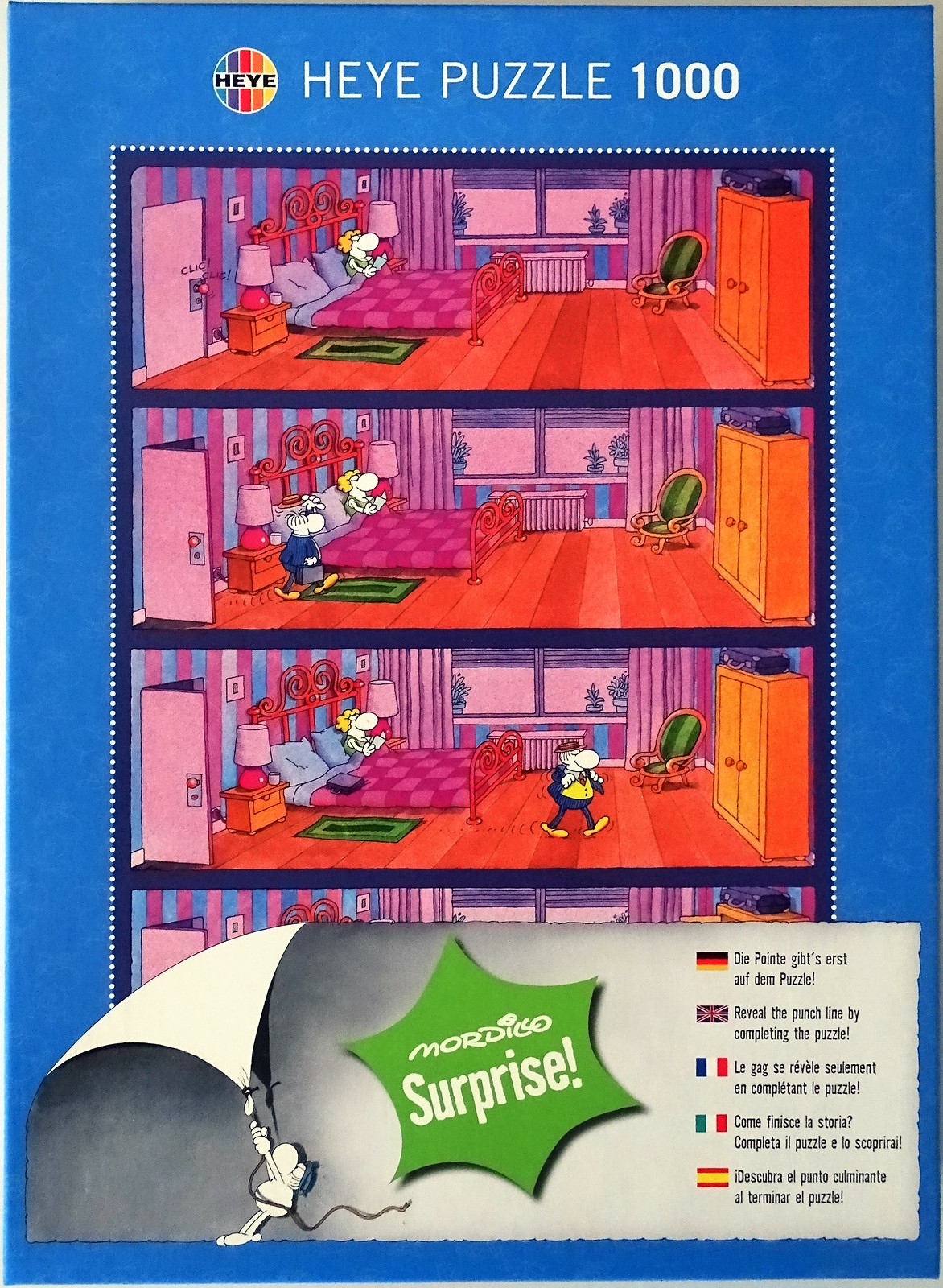This image depicts the colorful, comic-style cover of a "Heye Puzzle 1000." The cover features a prominent, thick, royal blue border, and at the top, in bold white letters, is written "HEYE Puzzle 1000" next to a circular logo with multicolored stripes and the letters "H-E-Y-E" in black. The central area of the cover displays a four-panel comic strip with a predominantly purple, blue, orange, and pink color scheme.

In the first panel, a cartoon woman with blonde hair is seen sitting in bed reading. In the second panel, her husband, depicted as an older man in a suit holding a briefcase, walks into the room. By the third panel, he is walking toward a dresser, unbuttoning his jacket. The fourth panel is obscured by a gray banner, which is being humorously pulled down by a small cartoon mouse wearing a blue hat.

Overlaying part of the image at the bottom is a green, starburst-shaped logo that reads "Mordeco Surprise!" in an excitable, vibrant font. To the right of the gray banner, various country flags, including those of Germany, Britain, France, Italy, and Spain, appear alongside text in multiple languages, presumably to advertise the puzzle. Additionally, some smaller cartoon characters can be seen in the corner of the image, adding to the lively and engaging design.